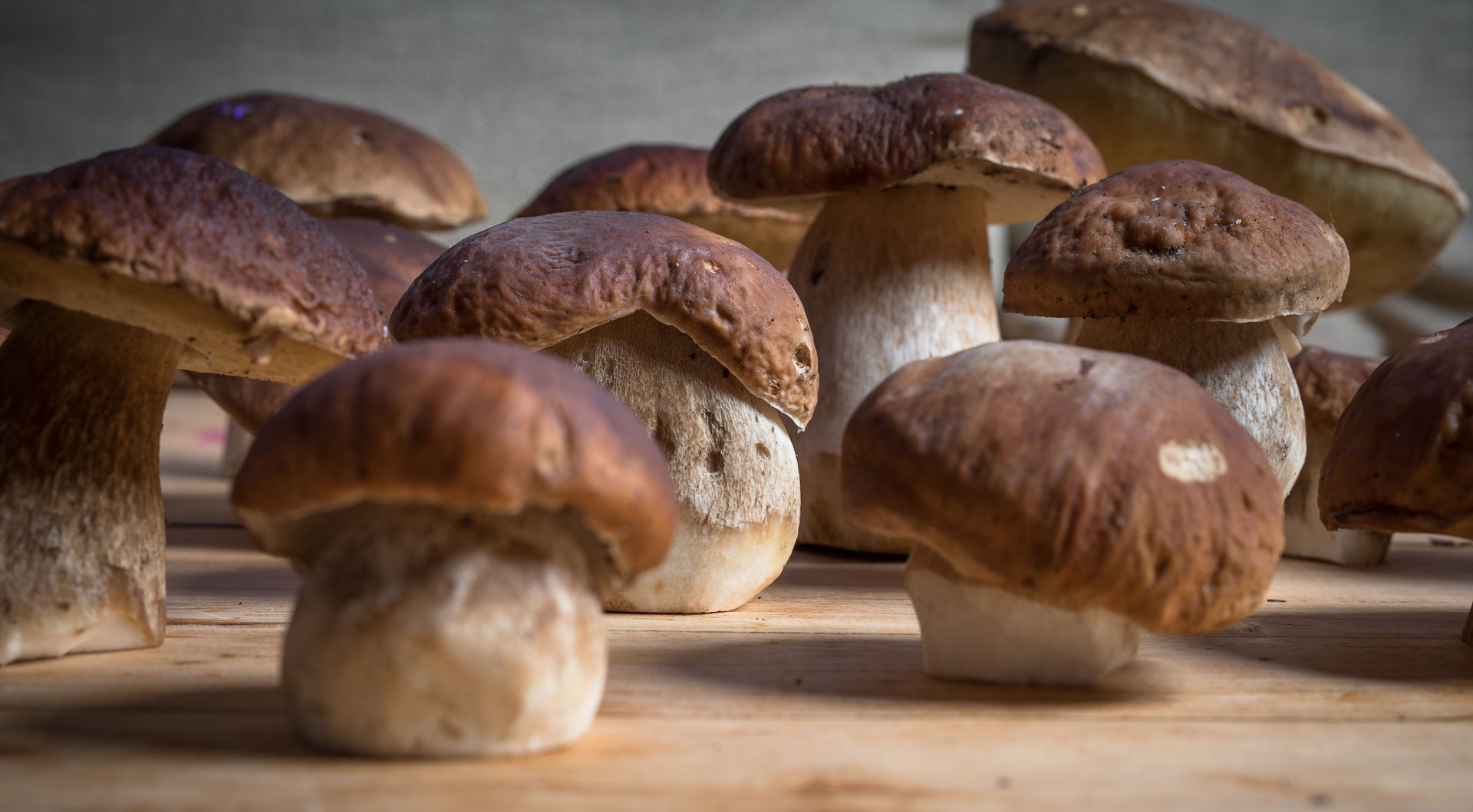In this image, a collection of approximately 15 mushrooms is displayed on a light brown wooden surface, which could be a table or a cutting board. The mushrooms exhibit a range of shades from light to dark brown, with some featuring distinctive purple accents and white bases. They vary in size and appearance, with the smaller, shorter mushrooms positioned in the front and the larger ones towards the back, including one particularly large mushroom in the far right with green accents on its cap. The mushrooms' tops are toasted and bumpy, suggesting age and a natural, imperfect texture. The background features a gradient of gray fading to black at either side, interspersed with lighter areas reflecting light. Shadows cast by the mushrooms enhance the depth of the scene, creating a natural and rustic aesthetic.